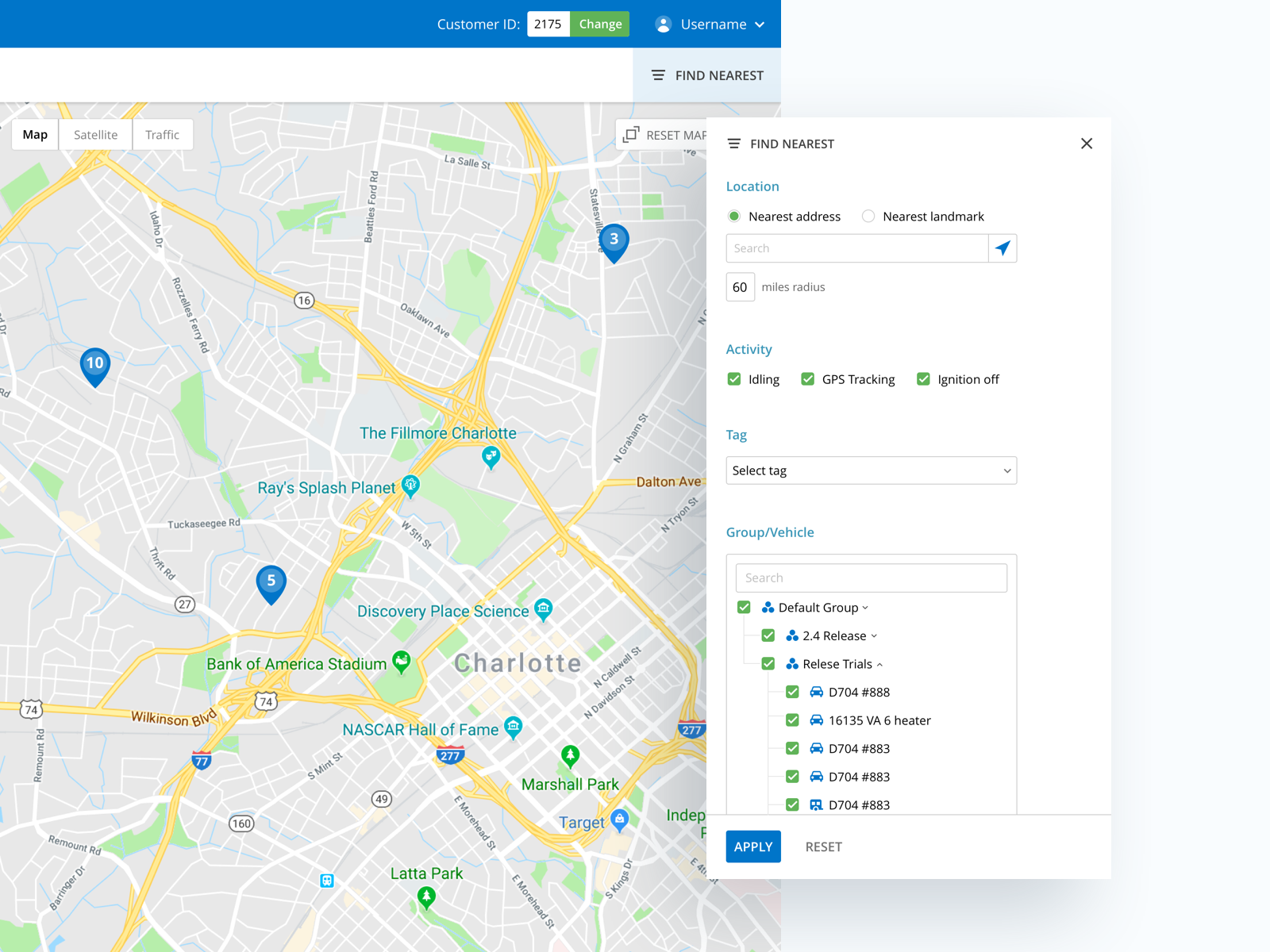This vertical image showcases a detailed user interface likely accessible via computer or smart device. The layout consists of a light grayish-blue sidebar on the right, a central white pop-up box, and a map positioned on the left. 

Across the top of the map section is a blue bar displaying "Customer ID: 2175" on the right, along with a green "Change" button. Nearby, a profile icon is labeled "Username," and below that is a "Find Nearest" option. The map itself appears to cover the area of Charlotte, highlighting various streets and landmarks.

The white pop-up box in the center focuses on the "Find Nearest" function, with an 'X' for closing the box in its corner. It offers options to search by "Location," "Nearest Address," or "Nearest Landmark," with "Nearest Address" currently selected. Below these options is a search bar with a filter set to a 60-mile radius. 

Additional activity filters— "Idling," "GPS Tracking," and "Ignition Off"—are all marked with green checkmarks. The pop-up also includes tagging options for "Tag," "Group," and "Vehicle." A default group with various selectable options appears, each accompanied by a checkmark box.